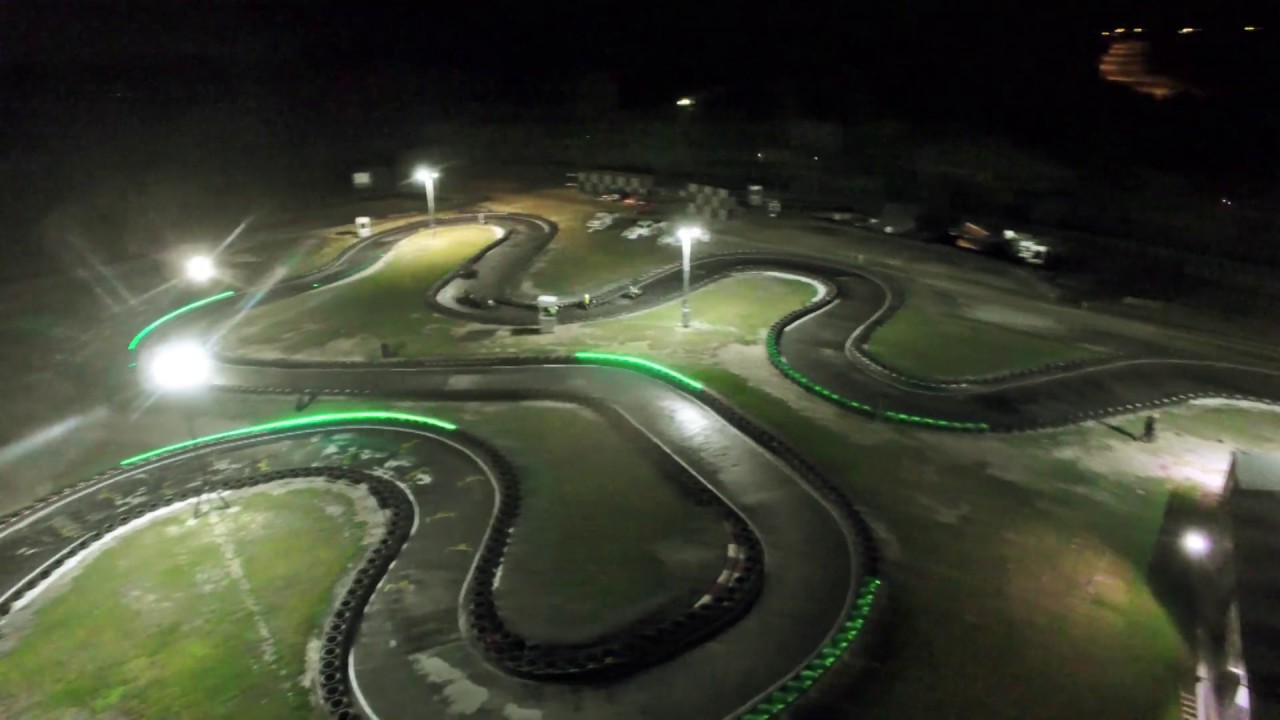The image captures an aerial nighttime view of a winding go-kart racing track, resembling the serpentine bends of a river. The track is made of dark concrete, glistening as though it has recently rained, and adorned with several green neon lines along the edges, highlighting its sinuous curves and S-shapes. Four to five street lights line the track, casting light onto the hairpin turns and the grassy central areas, ensuring the racers can navigate the course. Tires border parts of the track, especially prominent near a large curve in the foreground. The jet-black sky frames the scene, with a cluster of buildings and parked automobiles visible in the top right corner. Additionally, in the bottom right corner, there is a mechanized light machine, gray and white in color. Two go-karts are on the track, their drivers' helmets and gear reflecting the ambient light, adding a dynamic element to this meticulously detailed nightscape.